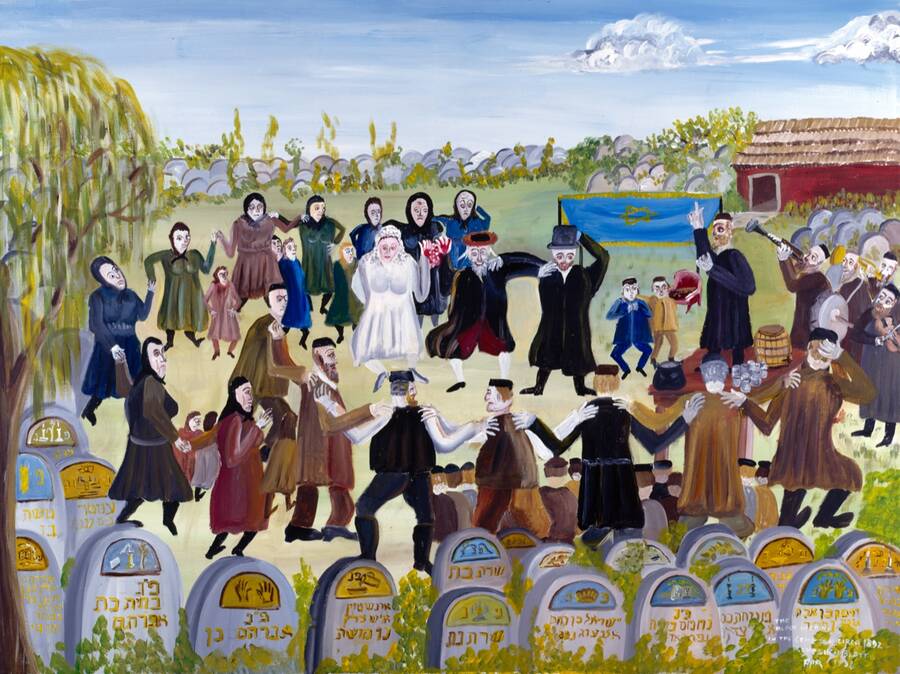This detailed painting depicts a vivid and conceptually striking Jewish wedding celebration set within a serene yet surreal landscape. Central to the scene is a woman in a white wedding gown, dancing amidst a circle of friends and family, all joyfully holding hands or linking arms as they move together. The diverse attendees include men wearing yarmulkes and top hats, along with a man in a distinct black robe, cranberry pants, white socks, and black shoes. Children also join in the festivities.

Musicians are positioned to the right with their instruments, adding a lively musical backdrop, while a small wine barrel with a spigot and a banner featuring a gold Star of David on a blue background enhance the celebratory atmosphere. The surroundings are unusual; gravestones with inscriptions in Hebrew encircle the lively group. In the background, a clear blue sky dotted with white clouds provides a peaceful contrast, flanked by a barn on the left and a tree to the right. The image is a blend of traditional celebration and contemplative elements, perhaps created with a brush, resulting in an evocative piece of conceptual art.